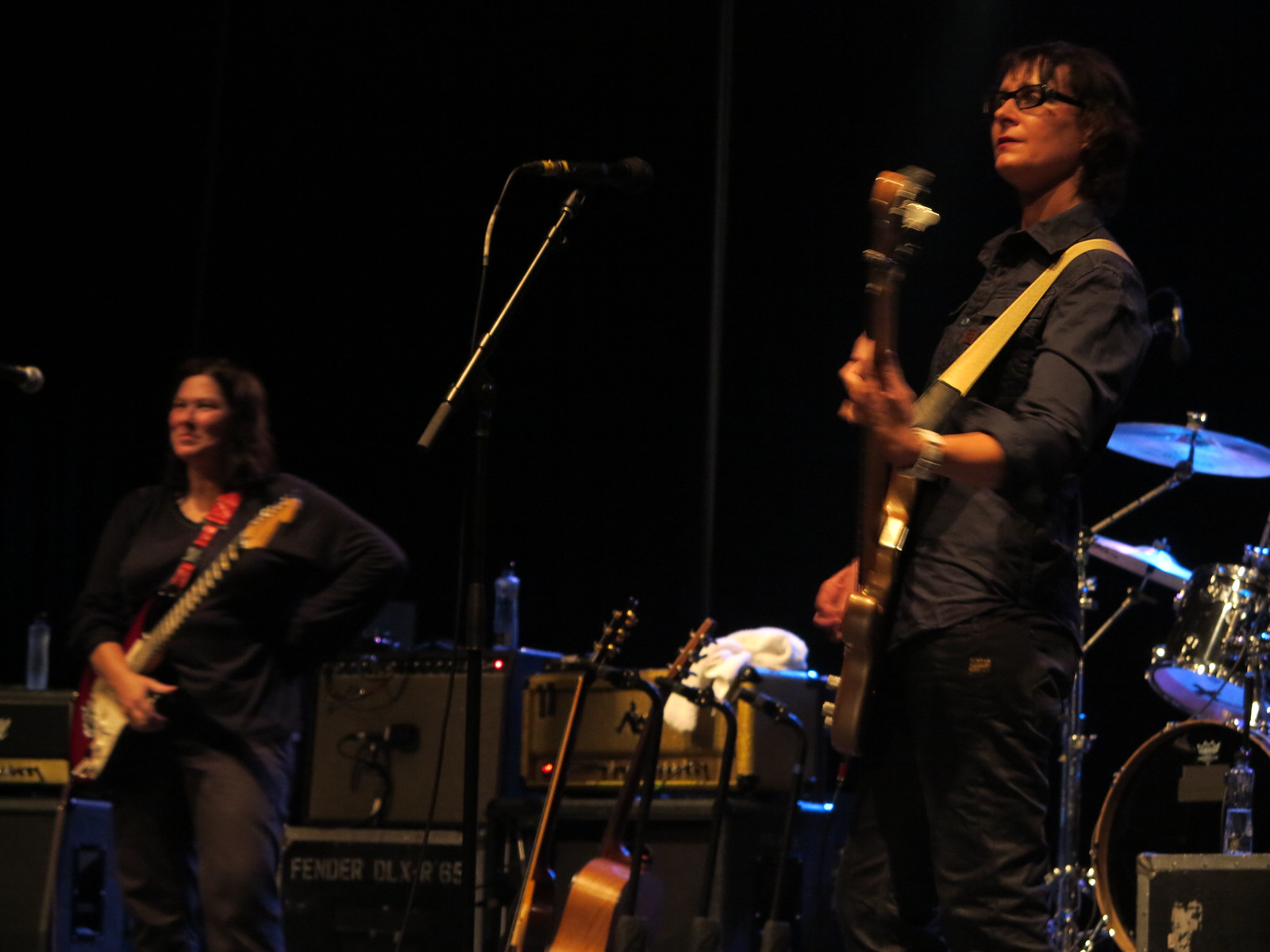The indoor photograph captures a live concert featuring a female band performing on a dimly lit stage with a dark background. On the lower left, a woman stands with her hand on her waist, smiling, and holding a red Stratocaster guitar; she wears a loose-fitting black top and black pants. To the right stands another woman, actively playing a bass guitar and wearing a black button-up shirt, black pants, and black rectangular glasses. Both musicians have microphones in front of them. The stage is equipped with various pieces of musical equipment, including a microphone, amplifiers, and guitar cabinets, along with leaned guitars against a railing in the middle of the photograph. An acoustic guitar and a black-neck guitar are also noticeable, as well as white towels placed on some of the amps. Behind the woman on the right is a partially visible black drum kit, complete with a cymbal. The overall scene exudes the energetic atmosphere of a night-time club performance.